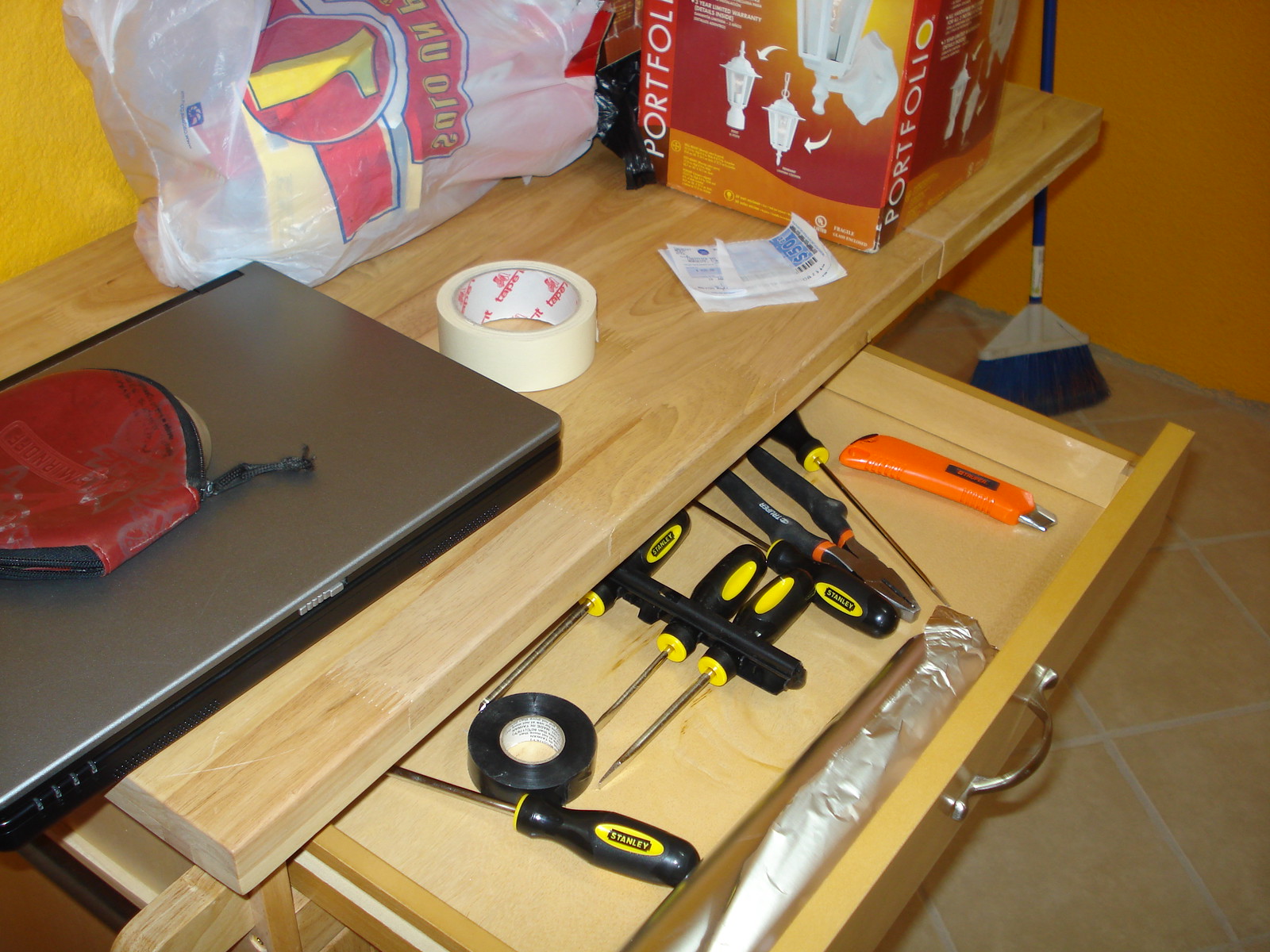A light golden wood desk, likely assemble-it-yourself, is prominently featured in the image. The desk, exhibiting the appearance of natural wood, has a top shelf and a lower section on the left with a pulled-open drawer. The drawer, which has a silver-tone handle, reveals a black holder containing three screwdrivers, and three more Stanley-branded screwdrivers, black with yellow, are scattered loosely within. Also in the drawer are a roll of black electrical tape, a pair of clippers with black handles, an unidentified bright orange tool, and a plastic bag.

On the top shelf rests what appears to be a somewhat thick silver-colored laptop with black sides. Adjacent to it is a round fabric bag with a black zipper, along with a roll of masking tape, a white plastic bag, and a box labeled "PORTFOLIO" that houses an outdoor white lantern, as depicted on the box. Completing the scene, a broom leans against an orange wall, set on a linoleum-covered floor.